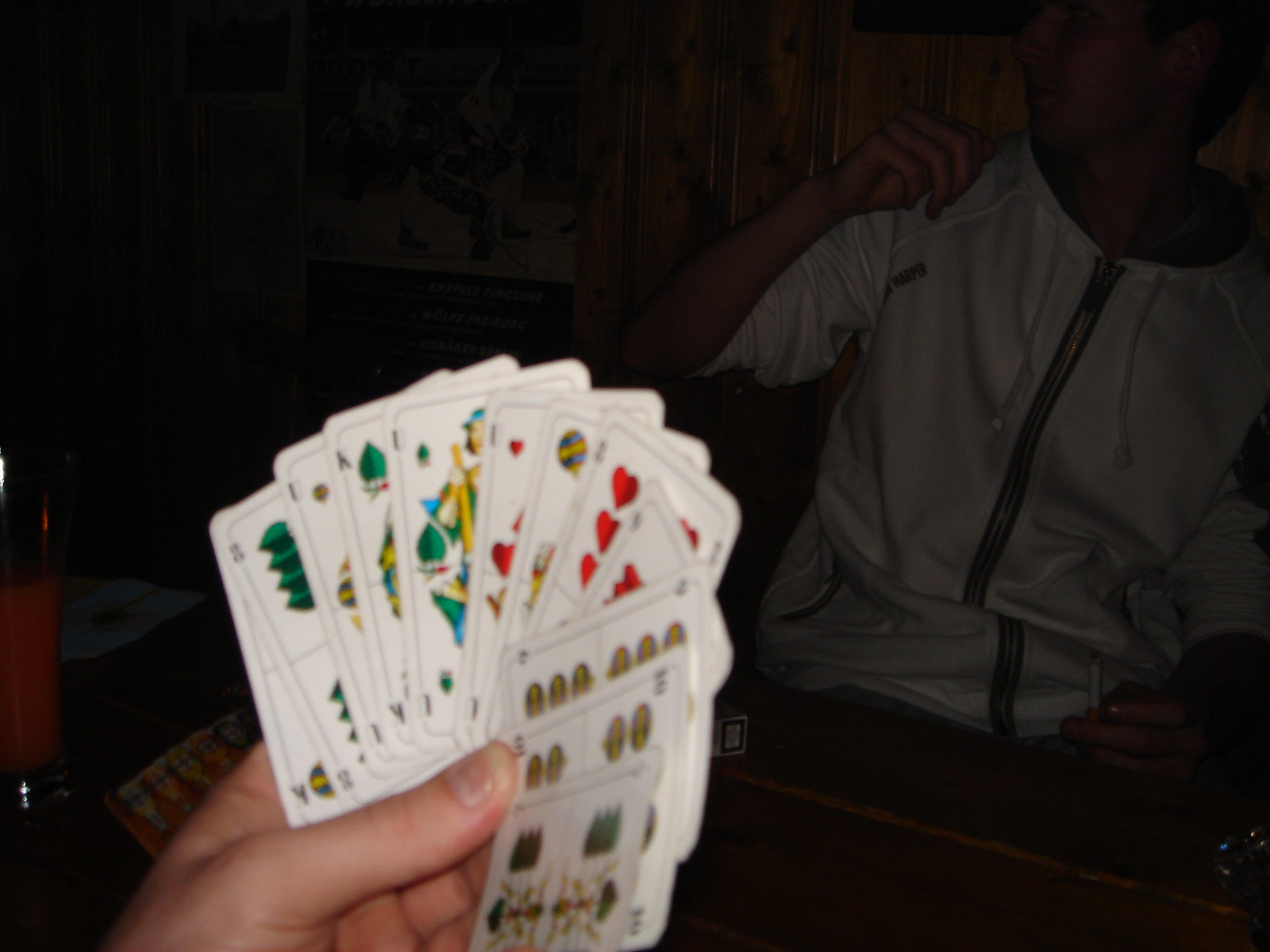The image features the hand of an unidentified individual, possibly belonging to a white person, as the hand's skin tone suggests. The hand, characterized by short nails which don't appear to be in the best condition, hints that it may belong to a man. The person is holding a collection of unusual, slightly blurred cards that deviate from a traditional deck. These cards are artistically styled, making them somewhat difficult to discern. Among the visible cards, there appears to be a three, a one, a king, another one, some hearts cards, a difficult-to-identify card, a two of clubs, and possibly an ace, summing up to over 10 to 15 cards in total.

To the right of the frame, a second hand is partially visible, likely belonging to another white individual. This person is clad in a white athletic shirt adorned with what might be drawstrings or dangling earbuds. The shirt features a zipper, indicating its casual nature. This second individual appears to be seated. The overall setting is dimly lit, suggesting an intimate, low-light environment where people are engaged in a card game.